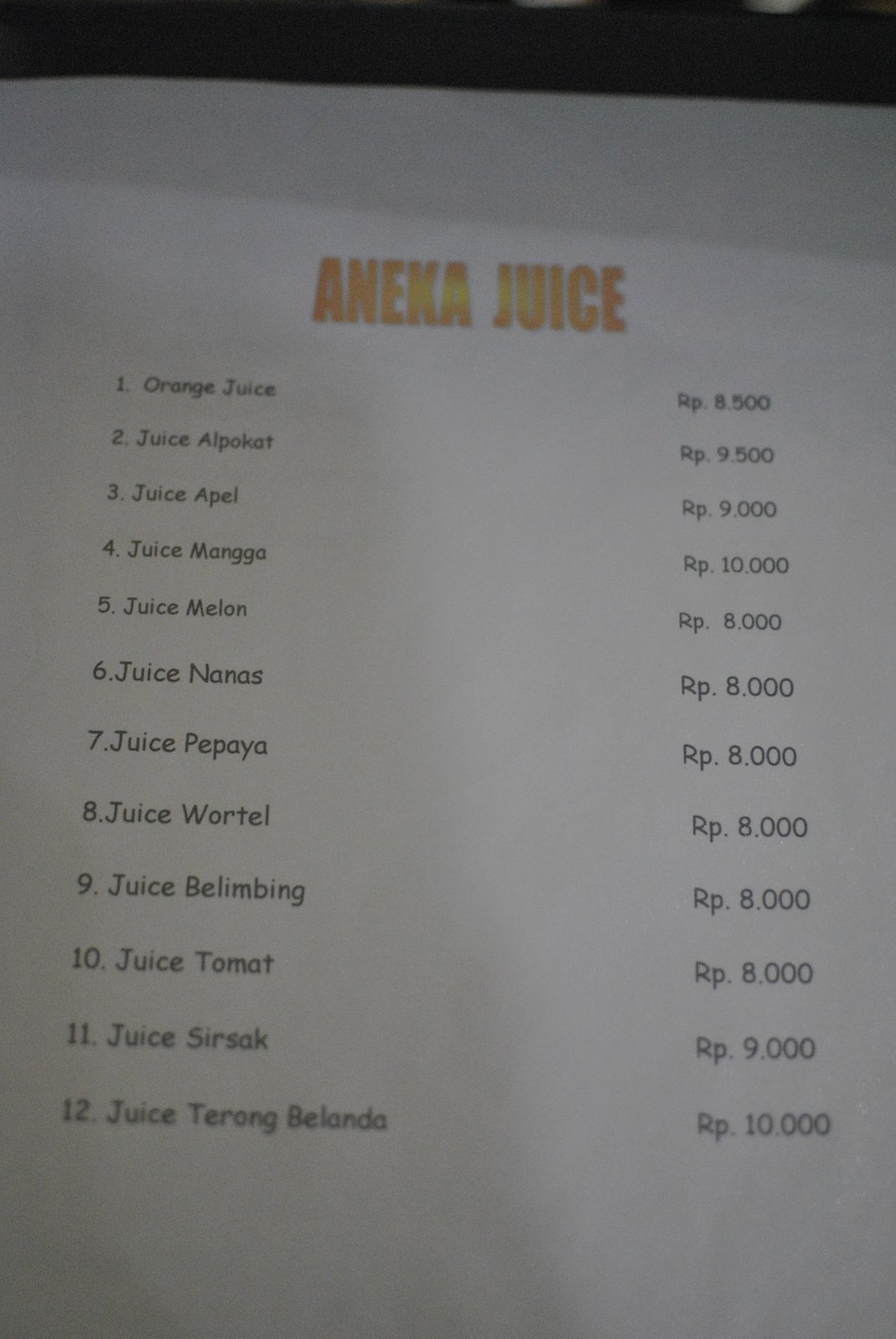This color photograph, taken in portrait orientation, captures a slightly grainy and low-light image, likely snapped by a smartphone in a juice bar. The focal point of the photo is a white sheet of paper featuring a juice menu under the vibrant, retro-styled header "ANEKA JUICE." The text, displayed in bold, capital letters reminiscent of 90s bubble-type writing, has an orange interior with a black outline and a yellow highlight running horizontally through the center. 

The menu lists twelve juice options, each associated with a number from 1 to 12 along the left-hand side. These options include both familiar and exotic flavors, such as Orange Juice, Alpokat, Tomat, and Sirsak. Each juice listing is followed by its price, formatted with a capital 'R' and lowercase 'p' (Rp), indicating a foreign currency. Prices are presented with three decimal points, e.g., Orange Juice at Rp 8.500 and Alpokat at Rp 9.500.

The image also captures slight shadows, suggesting the low-light conditions and the presence of the photographer. There is a distinct black bar at the top, along with shadows casting diagonally from the left towards the center right, likely from the person taking the photograph. The overall arrangement and details provide a clear view of an enticing and varied juice menu, reflective of a vibrant juice bar atmosphere.